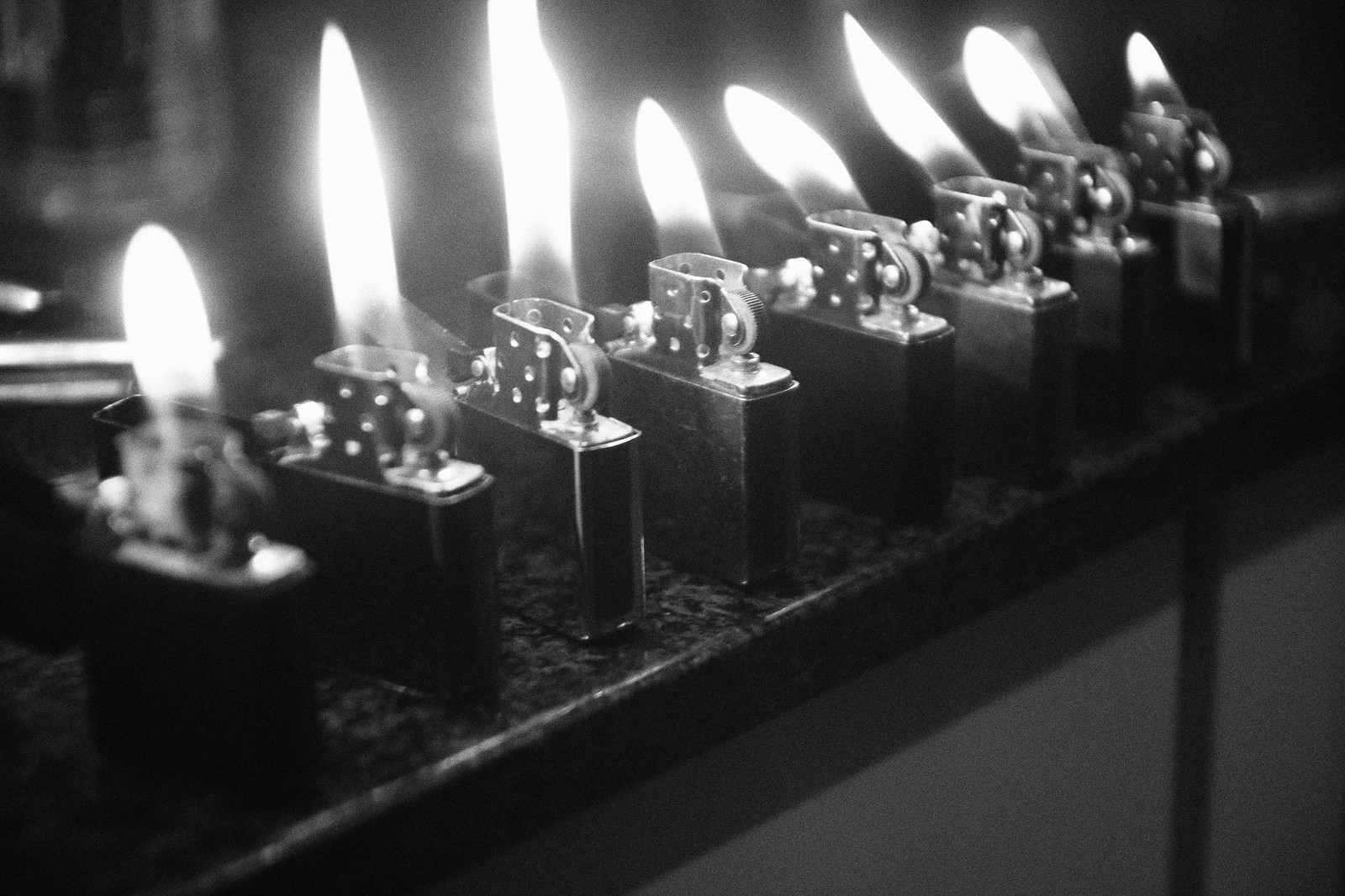This striking black-and-white photograph showcases a meticulously arranged row of eight vintage Zippo lighters, all uniformly open and aflame. The lighters are positioned diagonally across a sleek marble countertop, which extends from the bottom left to the center of the image, made of about one-inch thick granite. The Zippos, identical and spaced evenly, sit at the countertop's edge with their circular striker areas all facing the bottom left. Their silver tops catch the light, gleaming against the stark white flames and contrasting sharply with the dark background. Each flame varies in height, adding a dynamic element; the shortest flame is on the far left, while the tallest is the third from the left. Some flames appear to flicker as if caught in a breeze, enhancing the photograph's artistic appeal.